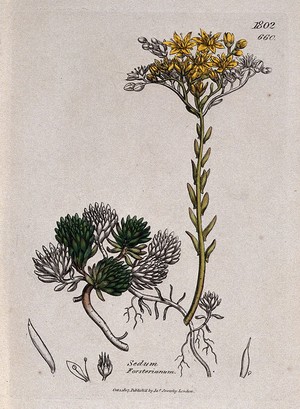The illustration features two distinct plants set against a white background, likely from a botanical field manual or textbook. The primary plant on the right extends from the bottom of the image to the top, characterized by a long green stem adorned with leaves and culminates in clusters of blooming flowers with yellow and white petals. The text "1802" and "660" are inscribed in the top right corner, and although there's text at the bottom middle, it's illegible. To the left of the main plant is a shorter, stout plant with dark green and white leaves, which some suggest might resemble a succulent. Both plants appear rooted in the same shallow base, with smaller green shoots emerging near the ground.